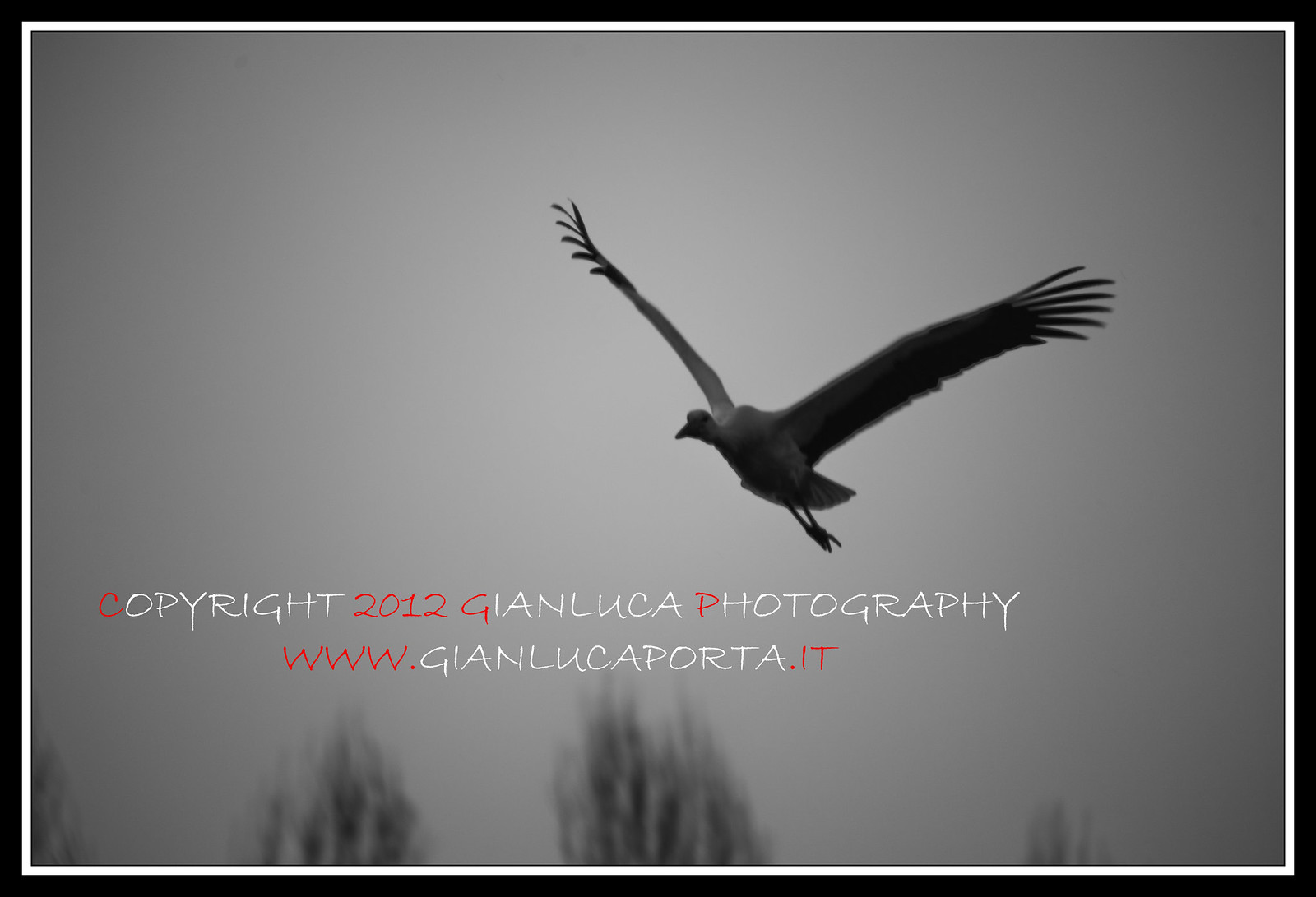A striking black and white, horizontally-oriented square image, framed by a black border and an inner white border. Dominating the center-right is a majestic large bird in mid-flight, its expansive wings arched upwards in a V shape, showcasing individual feathers, with those at the tips splayed distinctly. The bird's long neck extends downward, contrasting against its upward-printed body, while its beak, eyes, and black talons are clearly visible. The image is set against a backdrop of a gray gradient sky that lightens towards the middle. At the bottom, a few out-of-focus grayish trees and plants add depth to the scene. Overlaid text in mostly white, with specific red highlights, reads: “Copyright 2012, Gianluca Photography, www.gianlucaporta.it,” with the red highlights emphasizing the C of Copyright, 2012, the G in Gianluca, the P in photography, www., and .it.